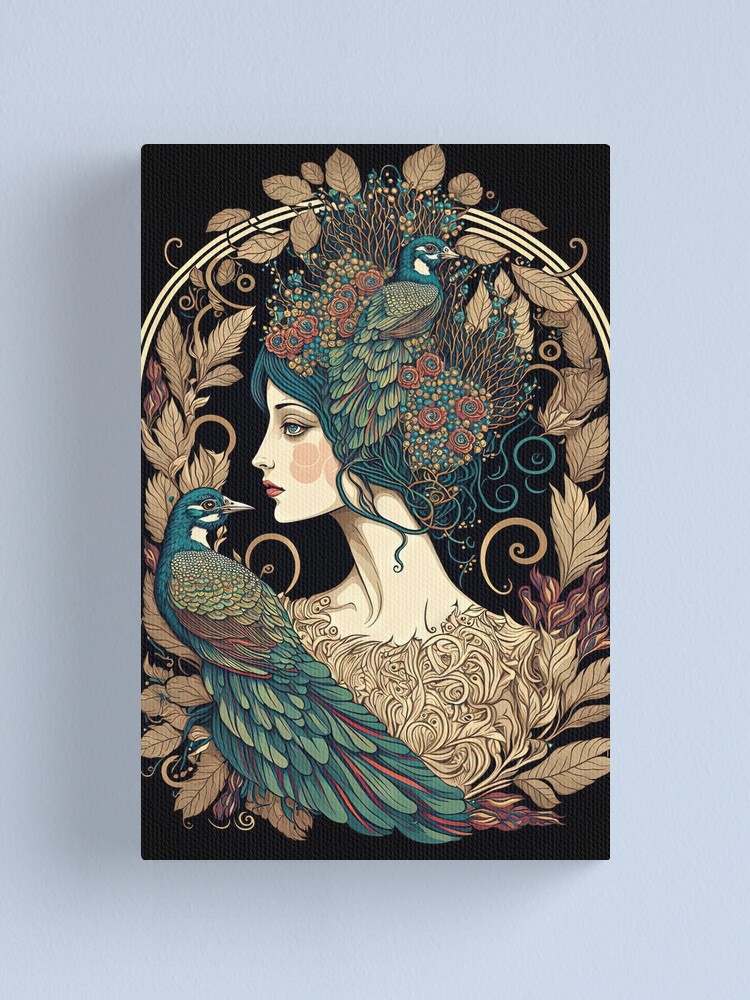This vibrant painting features a woman’s head and shoulders, set against a solid black background. Her hair, a lush green that swirls decoratively at the ends, is adorned with intricate floral designs and two striking peacocks. The peacocks, colored in hues of teal and red, with brown feathers and brown, sharply pointed beaks, merge seamlessly with her green locks. One peacock is positioned in front of her face, its beak nearly touching her chin, while the other is perched elegantly atop her head amid the floral arrangement. The woman faces to the left, with her face aligned closely with the front peacock’s beak. A half-circle arch in a light yellow hue adorned with golden brown leaves frames the upper part of the composition. Below, amber-colored leaves add to the natural motif. The entire image is set within a gray or bluish-gray background, reminiscent of the painting hanging on a wall. White lines near the birds' eyes add a touch of distinction to their expressive features.